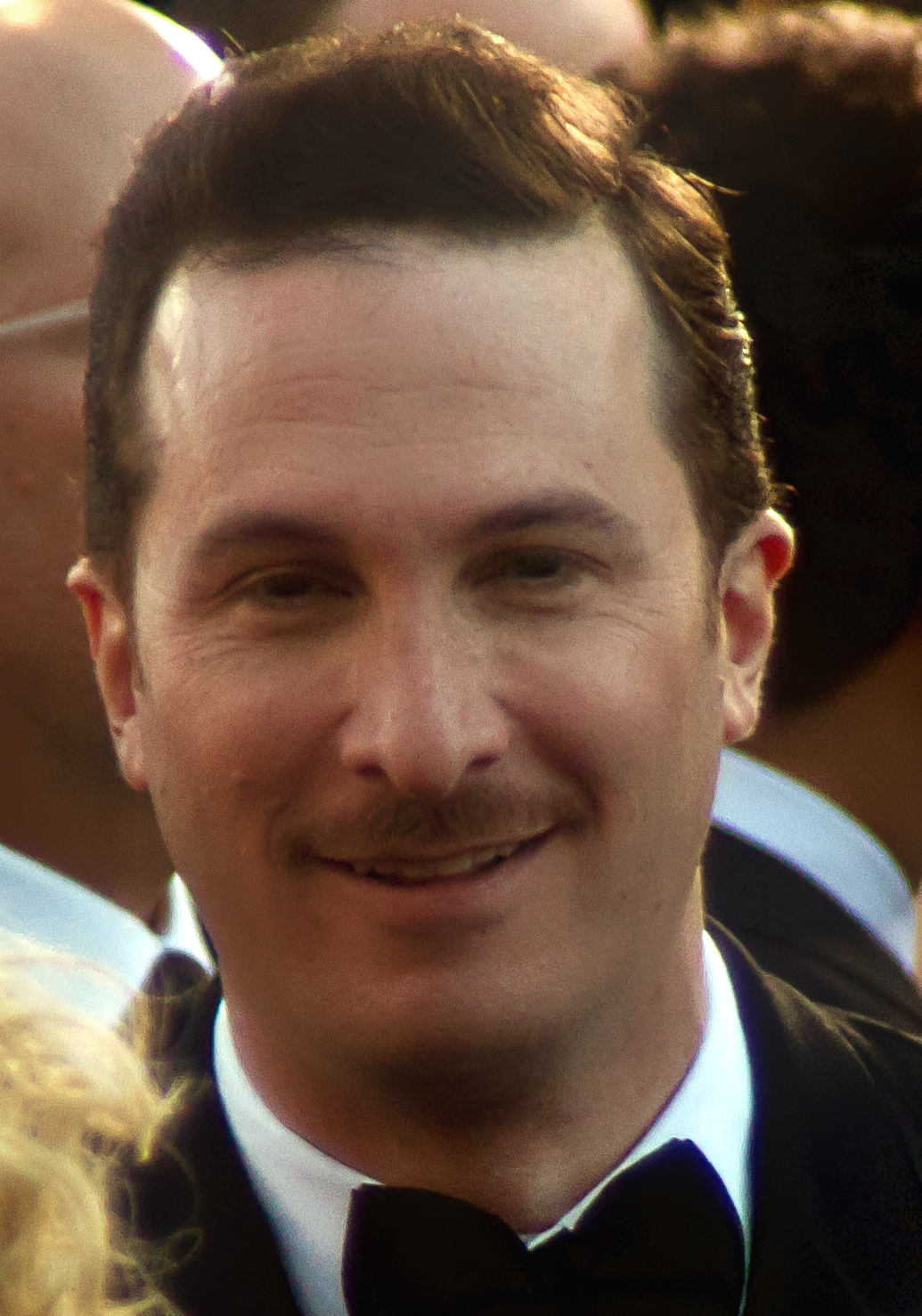The close-up photograph captures a well-dressed man centered in the frame, showcasing his upper shoulders to the top of his head. He sports a black tuxedo coat, a white formal button-up shirt, and a black bow tie. His short brown hair, swept back with a right-side part, accentuates his neat appearance. A mustache adorns his upper lip, and he gazes forward with brown eyes and a slight smile, revealing his upper teeth. His head is subtly cocked to the left. Surrounding him, the background features multiple out-of-focus individuals. To his immediate left, a bit of someone else's blonde hair intrudes the frame, while behind him, to his right, you can glimpse the back of another person’s head. Notably, two people wearing identical outfits stand to the far right, facing away from the viewer. The combined details emphasize the man's central presence amidst a bustling, partially obscured crowd.